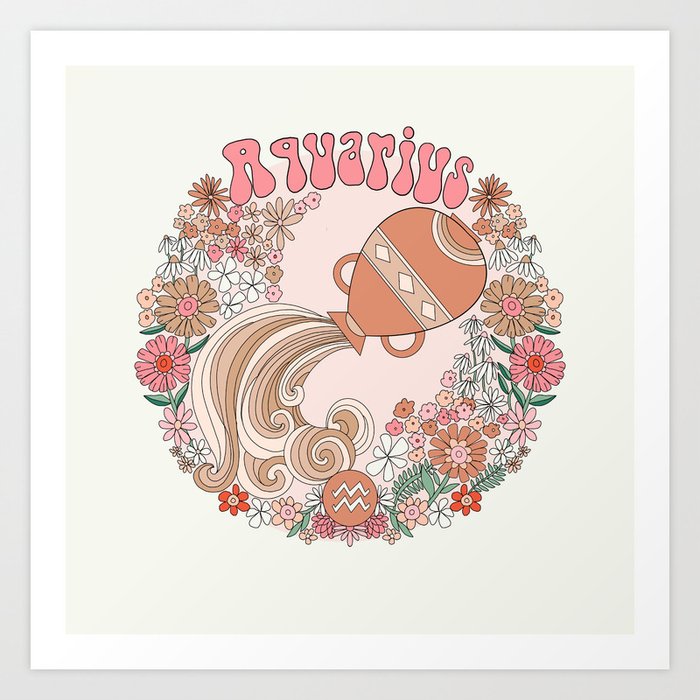This is a vibrant print of a colorful illustration titled "Aquarius" in a whimsical, '60s-inspired font. The square image is set against a light beige background with a white border and features a striking composition. At the center of the image, a ceramic jug adorned with geometric patterns spills out swirls of water, depicted in cream and light brown tones. Encircling the jug is a dynamic wreath of flowers, showcasing a cohesive palette of rust, tan, green, red, pink, and white. The overall effect is one of harmonious movement and playful energy, making it an ideal piece for decorating a bedroom or other personal space.